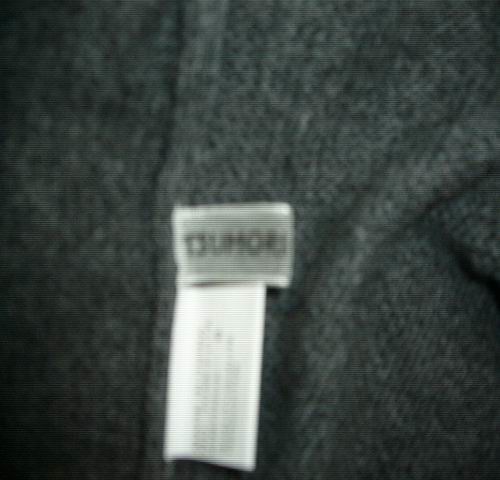This close-up image captures a section of dark gray knit fabric, likely from a sweater, with two tags sewn into its seam. The fabric appears slightly creased and bunched near the seam, indicating the garment is not laid completely flat. The primary tag is gray with similarly colored lettering that is somewhat blurry, presenting a possible inscription of either "D-U-M-O-R-S" or "D-U-H-O-R-S". Below this is a secondary, longer white tag that seems to contain care instructions, though the black printing on it is illegible.